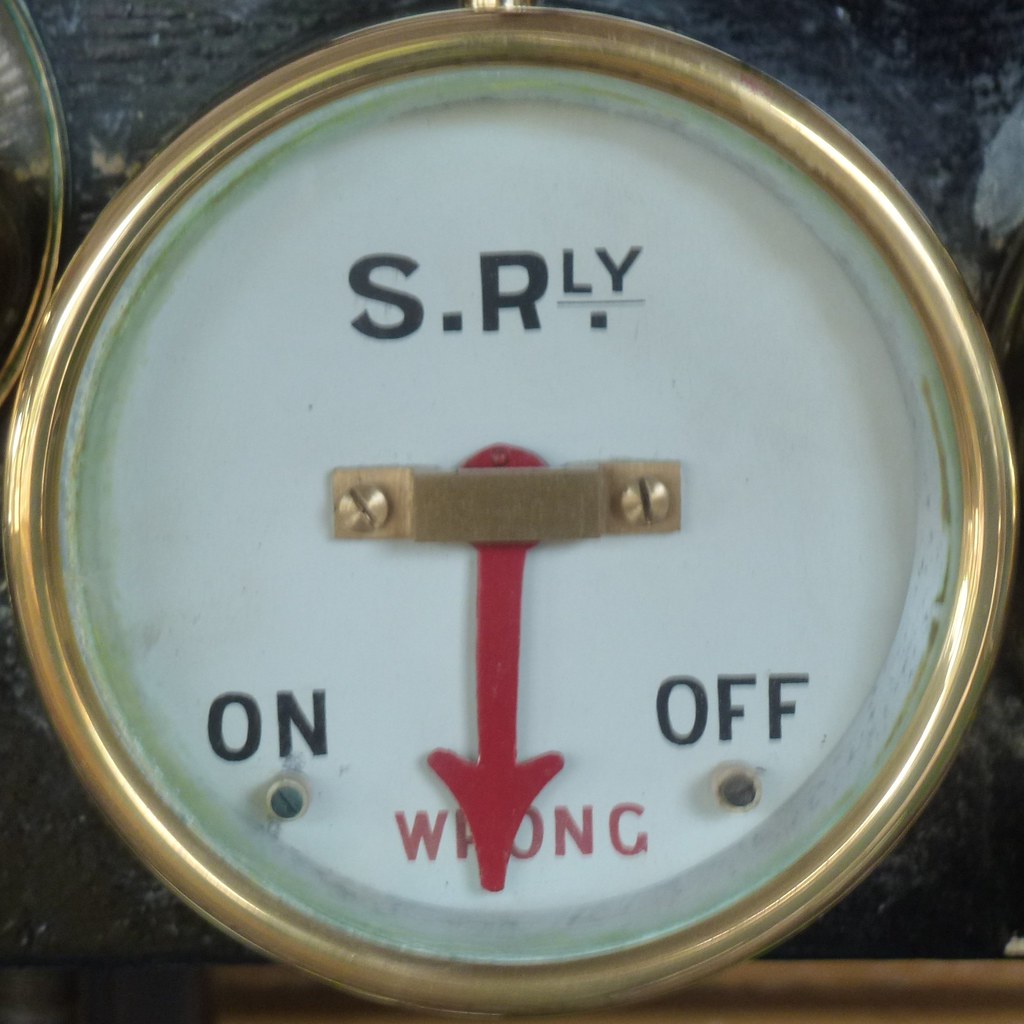This image is an extreme close-up, color photograph of a circular gauge or dial, possibly from old machinery, set against a fabric background with varied tones of dark gray and black. The dial is prominently positioned in the center of the frame and features a gold metal bezel. The background inside the bezel is white, and at the top of the gauge, it reads "S.R.L.Y." with the "L.Y." in superscript. In the center of the dial, a horizontal gold metal bar with two screws houses a prominent red arrow pointing directly downwards. Beneath this arrow, the word "WRONG" is boldly printed in red capital letters. To the bottom left of the gauge is the word "ON" in black, and to the bottom right, the word "OFF" in black. The image is clear and brightly lit, highlighting the contrasting colors of black, gold, white, red, and gray with photorealistic precision.